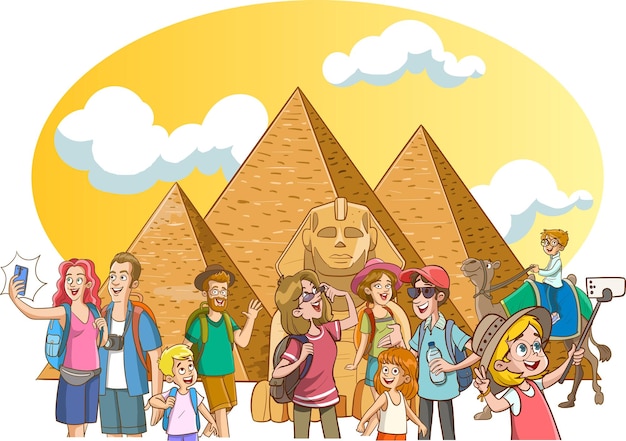In a vibrant, cartoon-style illustration, a lively group of tourists is depicted enjoying their visit to an iconic Egyptian landmark, with three majestic pyramids and the Sphinx forming a striking backdrop. The sky is ablaze with warm yellow hues, dotted by three fluffy white clouds, adding a touch of whimsy to the scene.

On the left side of the image, a young couple stands out. The woman sports vibrant red hair and is clad in a pink short-sleeved top paired with blue shorts. She accessorizes with a blue backpack and a fanny pack, all while capturing the moment with her cell phone, her face beaming with joy. Beside her, a young man dresses in a layered blue shirt over a white one, matching blue shorts, and has an orange backpack slung over his shoulders. He shares her smile as they immortalize their adventure in a photograph.

Next, a small blonde-haired boy grins happily, enjoying the moment. Near him is a middle-aged man donning a brown hat, green shirt, brown shorts, and a backpack. His glasses frame his bearded and mustachioed face, which looks straight at the viewer, radiating warmth and friendliness.

Beside him, a woman adjusts her sunglasses to get a clearer view, wearing a chic red shirt with white stripes on the neckline, sleeves, and hem, complemented by brown pants and a backpack. A little girl accompanies her, wearing a white tank top and orange shorts, her gaze fixed directly at the viewer with a wide, infectious smile.

Behind this small cluster is another couple. The woman is dressed in a pink hat, green shirt, red backpack, and blue shorts, standing alongside a man in dark sunglasses, a red baseball cap, a blue collared shirt, and gray pants. He carries a blue backpack and clutches a water bottle in his left hand.

Adding a playful element to the scene, a little girl wearing a brown hat and round glasses stands with a red tank top over a white shirt. She joyously flashes a peace sign with her right hand while expertly maneuvering a selfie stick with her other hand for the perfect shot.

Adding depth to the background, a young boy with glasses, riding a cheerful, smiling camel, grins widely at the viewer, completing the jubilant and dynamic tableau of tourists delighting in the timeless wonders of Egypt.